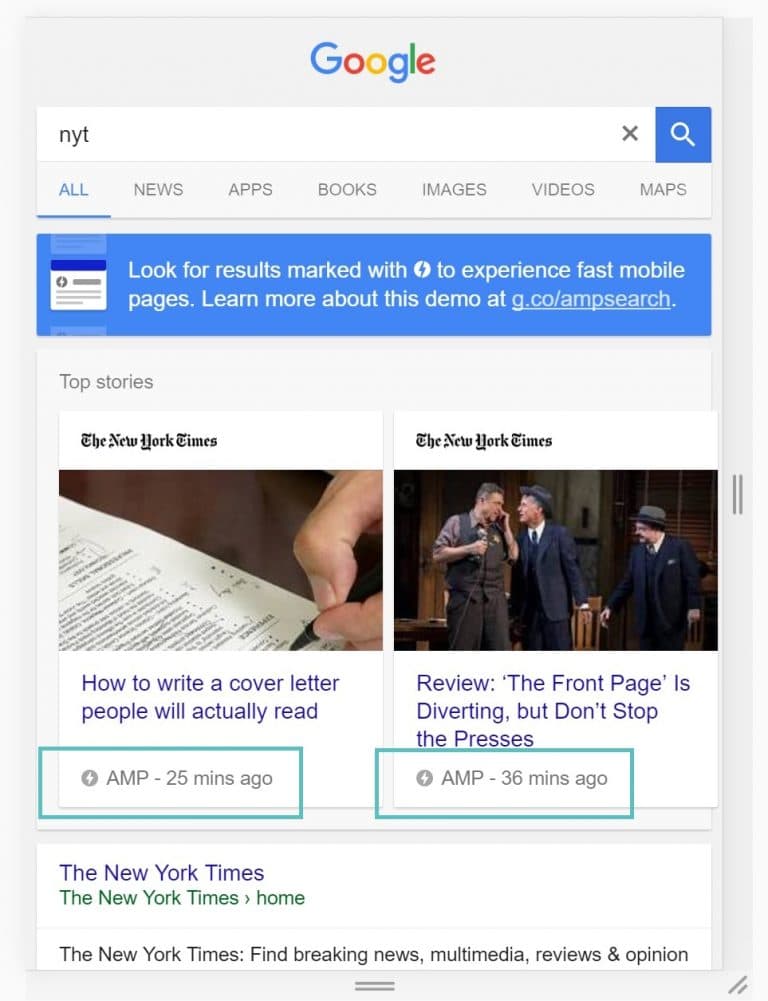The screenshot showcases a Google search page for "NYT," with the familiar Google navigation bar displaying options such as All, News, Apps, Books, Images, Videos, and Maps. Just below the search categories, there's a prominent blue rectangle advising users to "look for results marked with a lightning bolt to experience fast, mobile pages," and provides a link for more information at "g.co/amp-search."

Further down, there is a section titled "Top Stories" highlighted in white with gray text, featuring articles from The New York Times. 

1. The first article includes an image of a resume and is titled "How to Write a Cover Letter."
2. The second article is a review titled "The Front Page is Diverting, but Don't Stop the Presses."

Beneath these articles, there's a link to the New York Times website, providing quick access to their home page and content including breaking news, multimedia reviews, and opinions. The interface is completed with the recognizable Google logo in its traditional colors.